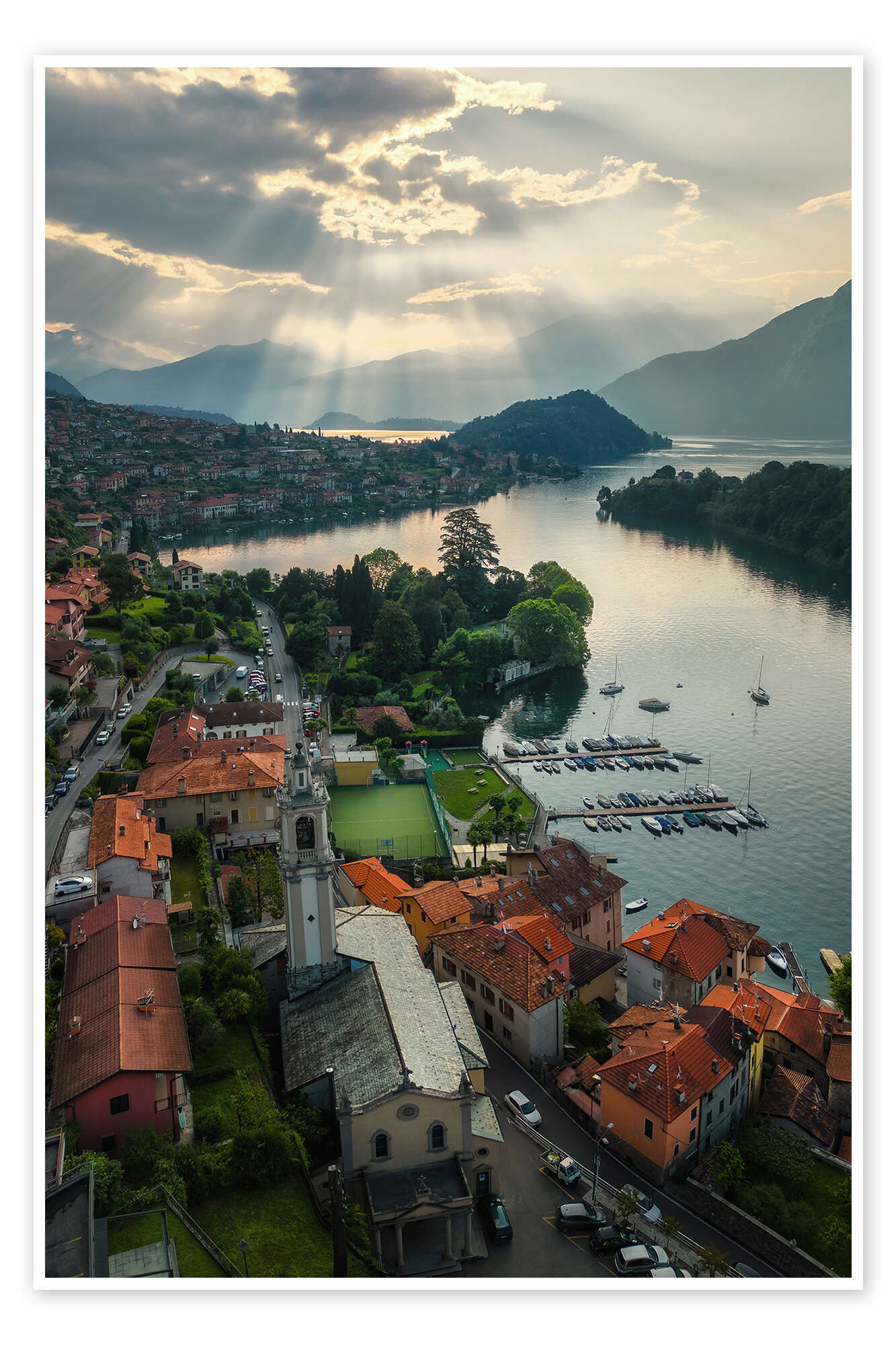This photograph captures a quaint, colorful lakeside town, likely European, set against an overcast sky with sunlight piercing through the clouds. The village, possibly Italian, features vividly painted houses with red tile roofs spread across a gentle hillside. A prominent tall church with a steeple stands out in the center, surrounded by various townhouses and slate-roofed buildings. A serene bay or inlet borders one side of the town, where a marina hosts an array of sailboats and other vessels, some docked and others floating freely. Cars are scattered along the charming, tree-lined streets that extend right up to the coastline. The background showcases forested hills and distant mountains, framing this picturesque, calm scene.